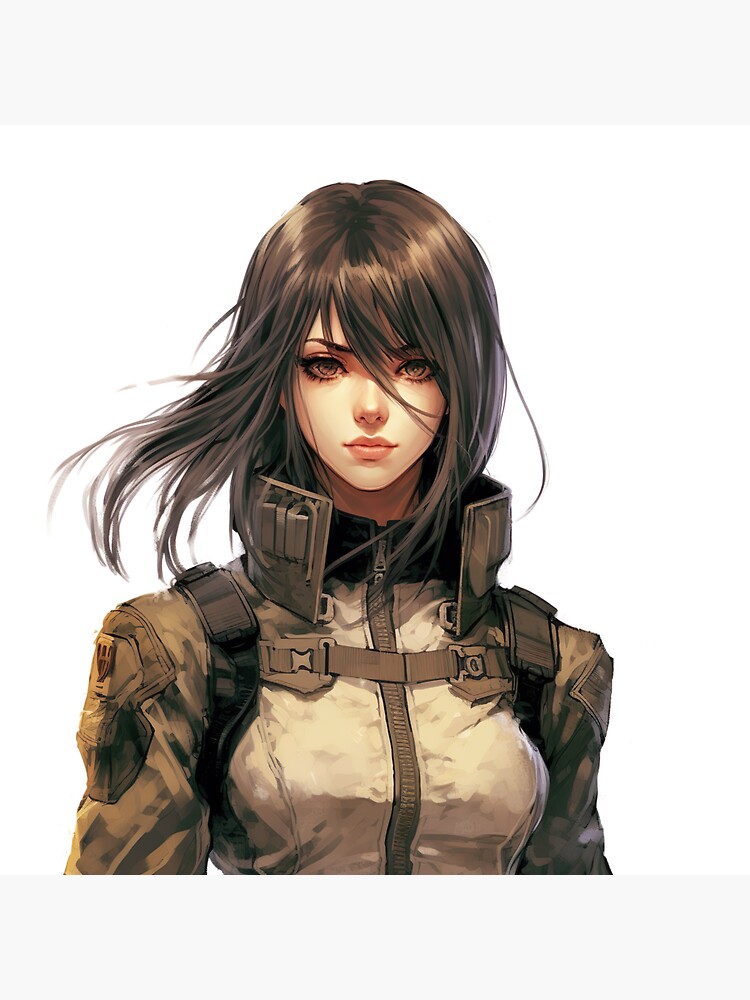The image depicts an anime-style female character, seemingly AI-generated, standing against a predominantly white background with a gray banner at the top. She faces the viewer with an intense, almost direct stare. She has a high-neck, military-style, tight-fitting jacket that zips up the middle, adorned with numerous clips, clasps, and patches on her arms. A clip secures the zipper at the top near her chest, and a hard collar with openings encircles her neck. The jacket's design suggests she might belong to a video game or anime series. She wears a backpack, with its straps visible across her shoulders and chest. Her long hair, a brownish-gray color with shaggy layers, flows as if swept by the wind from right to left. Her makeup accentuates her large, brown anime-style eyes framed by thick eyelashes and sharply defined eyebrows, while her lips are full and pursed, and her pointy nose and chin complete her expressive face. She has fair skin, and her overall appearance combines a sense of elegance and strength.